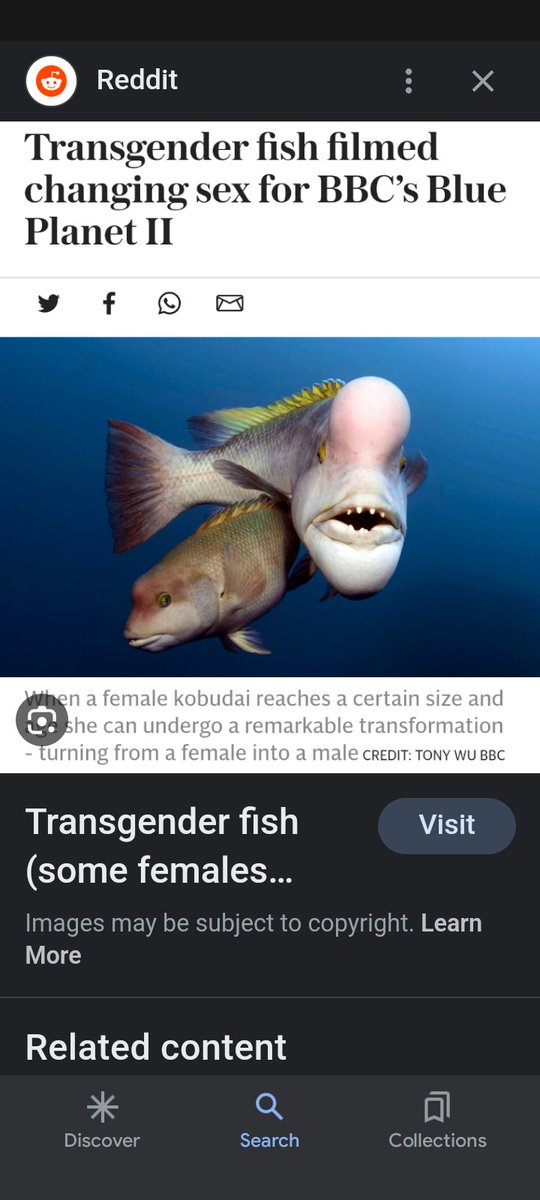This is a detailed caption describing the screenshot of the Reddit app interface:

---

The screenshot showcases the Reddit app interface on a mobile device. At the top left corner, the iconic Reddit logo is prominently featured, consisting of a small white alien figure set against an orange circle. Directly beside it is the text "REDDIT" in capital letters. The top banner is minimalist, featuring the black Reddit symbol, a set of three dots for settings, and a white "X" for closing the app.

The main content displayed appears to be a preview of an article shared within a subreddit. The article is titled "Transgender Fish Filmed Changing Sex for BBC's Blue Planet 2." Accompanying the shared article are icons for sharing the content via Twitter, Facebook, WhatsApp, and email.

The preview text of the article reads: "When a female kobudai reaches a certain size and [partially obstructed by the Canberra logo] she can undergo a remarkable transformation, turning from a female into a male."

Below this text is the subreddit post title, "Transgender Fish," followed by partially visible text in parentheses: "some females..." due to an ellipsis indicating it has been cut off. 

On the right side, there is a "visit" symbol, indicating that this Reddit page has not been selected yet but is visible in the search results. Below this, the interface suggests related content; however, the visible part of the screenshot ends there.

At the bottom of the screen, a navigation bar lists three options: "Discover," "Search," and "Collection," implying that the screenshot is likely taken from within a search engine app.

---